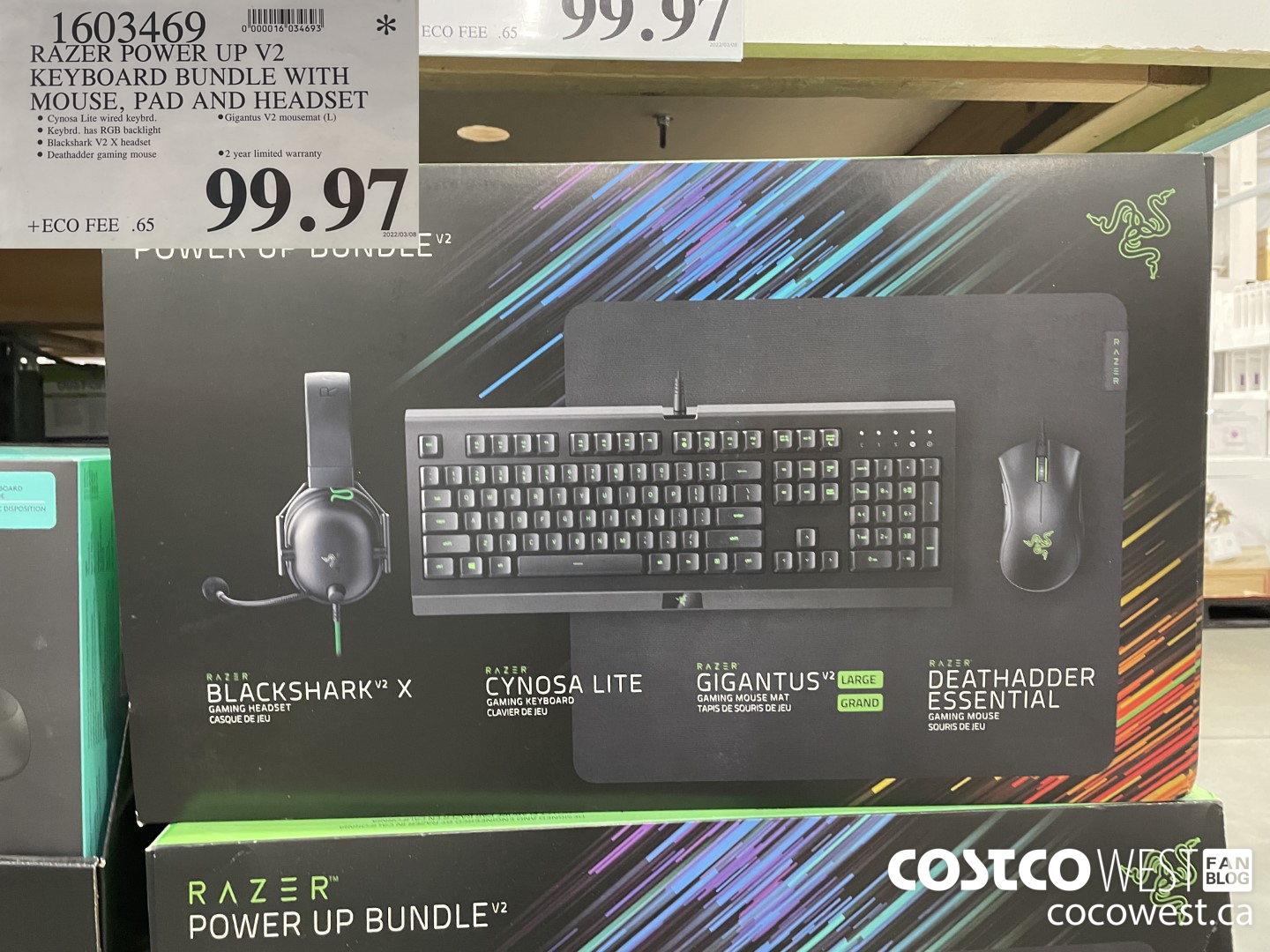The image showcases a Razer PowerUp V2 Keyboard Bundle on display at a Costco store. In the top left corner, there is a large white square tag detailing the bundle's contents, which includes a keyboard, mouse, mouse pad, and headset. The tag specifically reads: "Razer PowerUp V2 Keyboard Bundle with Mouse, Pad, and Headset."

The bundle is housed in a large black box prominently displayed atop another box. The top right corner of the packaging features the distinctive Razer logo. Centralized on the front of the box are images of the included products, each accompanied by a description.

On the box's left side, there is a side view of the headset labeled "Razer Black Shark X Gaming Headset." In the center of the box, you can see the keyboard termed "Razer Cynosa Lite Keyboard," along with the "Razer Gigantus V2 Gaming Mouse Mat" positioned below it. On the far right side of the box, the included mouse is labeled "Razer Deathadder Essential."

Additionally, the bottom right corner of the image features a price tag indicating the bundle costs $99.97 in US dollars. Also in the bottom right corner, there is a watermark that reads "Costco West Fan Blog."